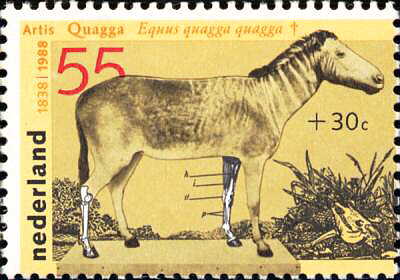The image depicts a commemorative stamp from the Netherlands celebrating the 150th anniversary with dates "1838-1988" displayed vertically on the left side. The main image showcases a quagga, a now-extinct zebra variant with the Latin name Equus quagga quagga, featuring a zebra-like neck and a horse-like body. The animal is tilted sideways and facing right, with labels and arrows pointing to its legs, highlighting areas with distinct black and white coloring. In addition, there is text at the top that reads "Artis Quagga, Equus Quagga Quagga." The stamp also includes a large "55" indicating its cost, and another marking "plus 30 C" on the right. At the bottom right, you can see a patch of grassy terrain with a quagga skull nestled in it, adding a poignant detail to the imagery.